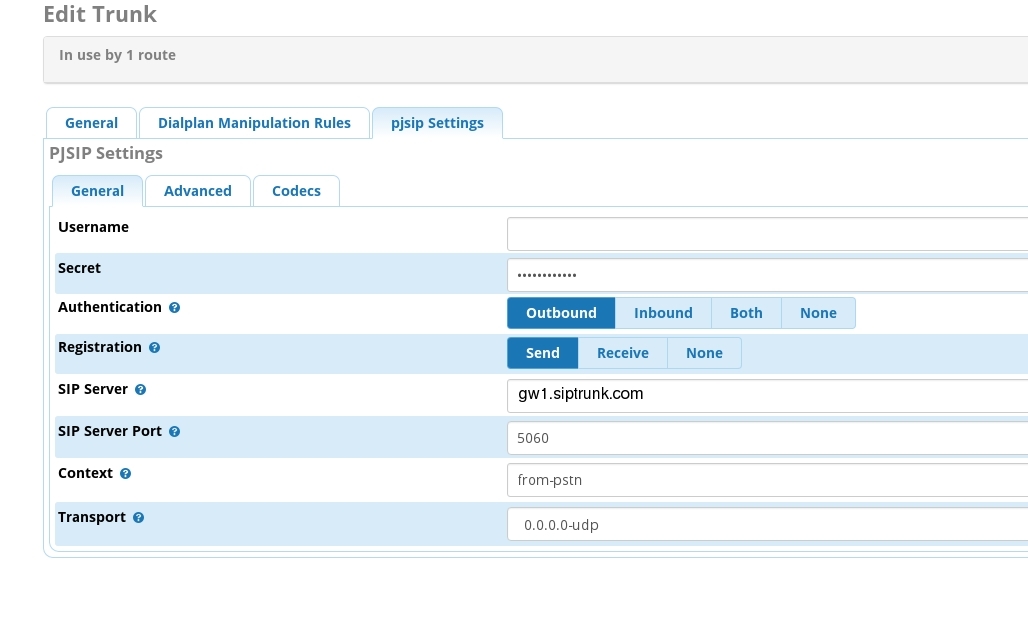This detailed screenshot captures a computer settings interface, specifically focusing on configuring a trunk. At the top, in gray text, the heading reads "Edit Trunk" with a subheading below it stating "In use by one route." 

The interface is divided into several navigational tabs, all in blue text. The tabs include:
1. General
2. Dial Plan Manipulation Rules
3. PJSIP Settings (highlighted)

Within the "PJSIP Settings" tab, there are three sub-tabs, also in blue text, labeled:
- General (highlighted)
- Advanced
- Codecs

In the "General" sub-tab under "PJSIP Settings," the options and fields are presented in black text:

1. **Username**: A white entry box to the right of this label.
2. **Secret**: Displayed as dots within a window to protect the hidden information.
3. **Authentication**: Options include Outbound, Inbound, Both, and None, with Outbound highlighted in dark blue and white text.
4. **Registration**: Options include Send, Receive, and None, with Send highlighted in dark blue and white text.
5. **SIP Server**: The text box to the right contains "gw1.siptrunk.com".
6. **SIP Server Port**: The entry box contains the default port number "5060," appearing shaded.
7. **Context**: The text box to the right reads "From-PSTN".
8. **Transport**: The box to the right displays "0.0.0.0.UDP".

The fields for "Secret," "Registration," "SIP Server Port," and "Transport" are all highlighted in light blue, indicating they are currently editable or focused.